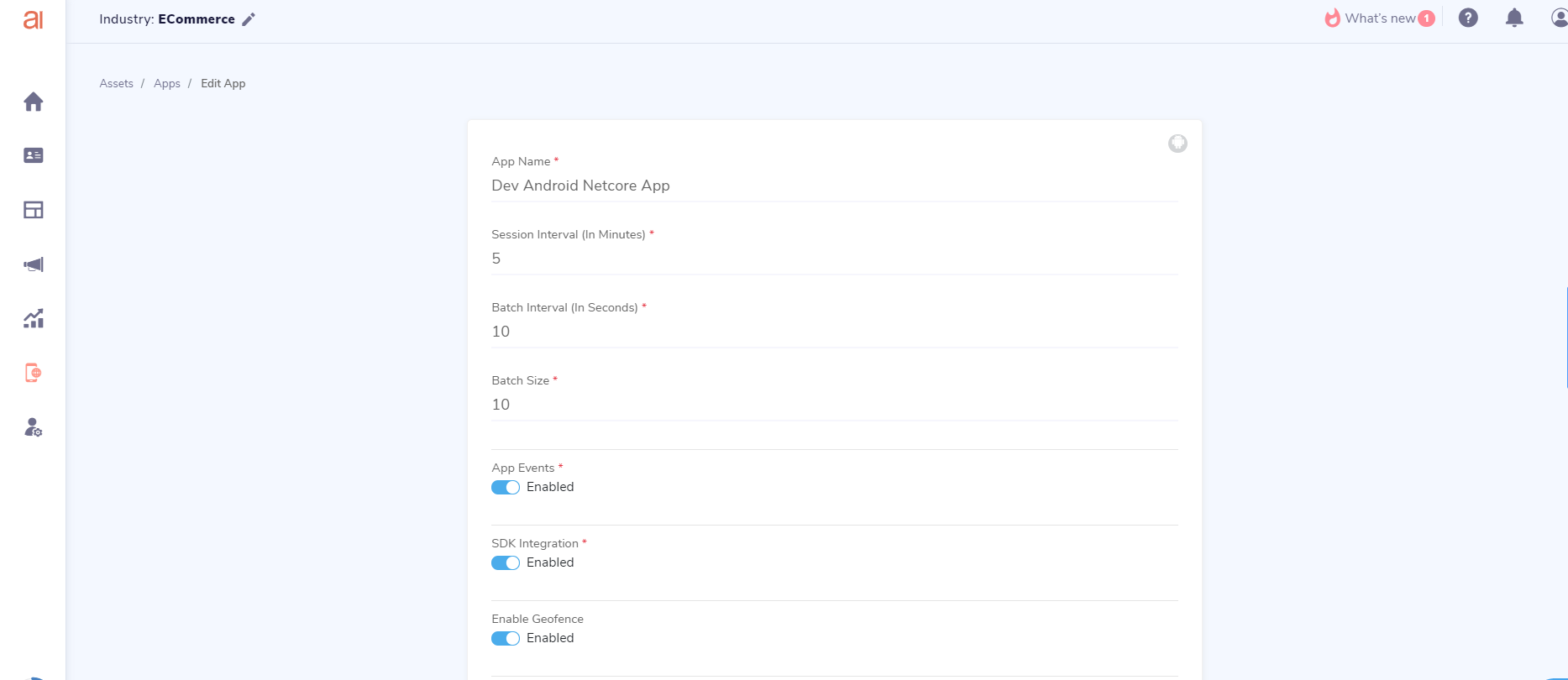The image depicts a detailed user interface (UI) likely related to an e-commerce or industry-specific application, with a focus on artificial intelligence (AI). The main screen features a home icon and a series of other icons used for page layout, displaying graphs, and various functionalities. 

On the left side, beneath the AI label (written in lowercase letters), there are seven icons. These likely represent different sections or tools, such as Assets, Apps, and an Edit App option. Additional labels include "What's New," a bell icon for notifications, and a human face icon, presumably for user account or profile access.

In a central panel or section, there's a list titled "Assets/Apps/Edit App," which includes details about specific applications. Examples include an app named "Dev Android Net Core App," though some of the text is unreadable. Beneath this title, there’s a number five, followed by more text and a number ten, possibly indicating batch sizes. This section also features "App Events Enabled" with an active blue toggle switch, suggesting that these events are currently enabled.

Additionally, there’s an SDK (Software Development Kit) integration, indicated as being enabled, along with other unreadable options that are also enabled. In the upper-right corner, a prominent "What's New" feature is highlighted with a pink fire icon, followed by an exclamation mark. Adjacent to this, there is a question mark inside a circle, a bell icon, and a human face icon, suggesting additional notifications or help options.